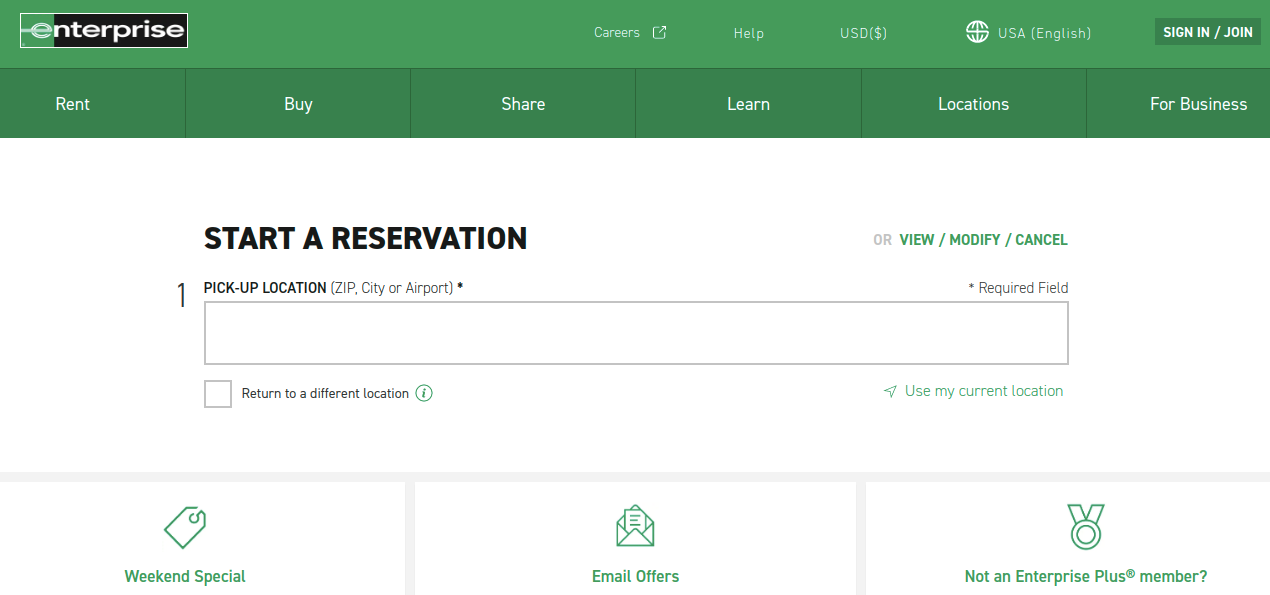The image captures the Enterprise Rent-A-Car website interface. At the very top of the page, there is a horizontal light green rectangle, beneath which lies a darker green rectangle. Starting from the top left corner, the 'Enterprise' logo is prominently featured. The logo displays a white 'E' with a light-colored background, followed by the letters 'N-T-E-R-P-R-I-S-E' in white on a black background.

Moving towards the center-right area, there is a clickable 'Careers' link accompanied by an icon of a diagonally right-pointing arrow. To its right, there's a 'Help' link followed by a currency selector marked as 'USD ($)'. Continuing to the right, a small icon of a white globe is visible, with text next to it indicating 'USA (English)'. Further right, there is a dark green 'Sign In / Join' button with white letters.

Below this section, in the darker green area from left to right, are white text buttons labeled 'Rent', 'Buy', 'Share', 'Learn', 'Locations', and 'For Business'.

Beneath this menu, bold black letters spell out 'Start a Reservation', accompanied by the word 'Or' in gray, and 'View / Modify / Cancel' in green text. Below 'Start a Reservation', there are instructions for specifying a 'Pickup Location' with an example of 'Zip, City, or Airport' noted in small black letters.

A search bar is placed underneath this instructional text. Below the search bar, there is an empty gray checkbox next to the text 'Return to a different location'. To the right of this checkbox is a circle with an exclamation point inside it, and to the far right, a diagonally upward facing arrow followed by the text 'Use my current location' in green.